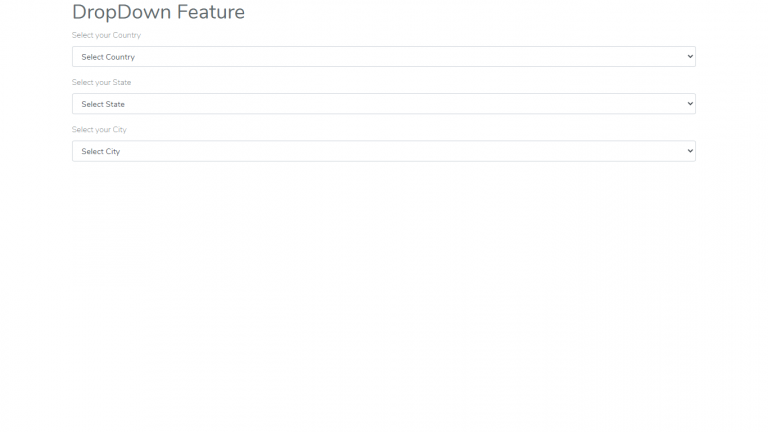This black-and-white screenshot features a user interface from an unidentified website, showcasing a dropdown selection functionality at the top. The interface prompts users to choose their geographical location in a sequential manner, starting with "Select your country," followed by "Select your state," and concluding with "Select your city." Each prompt is accompanied by a dropdown arrow box for making the selection. The image is predominantly textual, formatted in a landscape orientation, with no visual elements such as photographs, illustrations, people, animals, plants, or machinery.